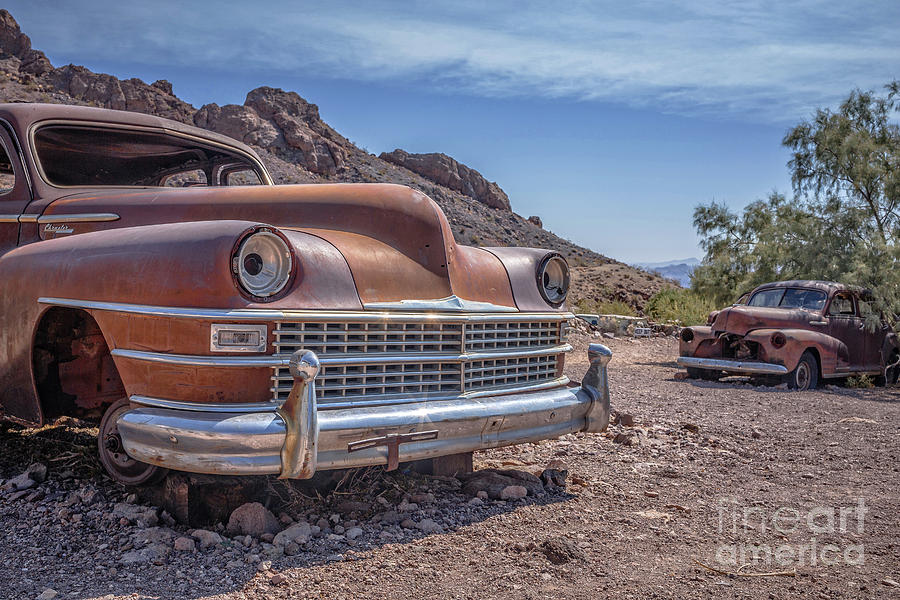In this striking photograph, two abandoned classic cars, reminiscent of the big-bodied, round-hooded designs of the 1950s, sit in a sparse desert landscape beneath a vivid blue sky streaked with high white clouds. Dominating the background is a rugged, bare mountain with large beige and brown rock outcroppings leading into distant rolling hills. The ground is strewn with various-sized rocks and dirt, devoid of vegetation except for a full-leaved deciduous tree partially enveloping the car on the right and two small green bushes nearby.

The car on the left, closer to the foreground, is an orange Chrysler, identifiable by its emblem, resting on blocks with no wheels. Its headlights lack bulbs but retain their characteristic silver housing. It has a complete front bumper, additional lower lights, but is missing the windshield and a license plate. The car on the right, in worse condition, has a missing headlight housing, an absent front bumper but an intact lower front bumper, and is more heavily rusted than its counterpart. Its windshield remains intact, though it lacks silver reflective license plate housing.

This visually arresting scene, with its juxtaposition of decaying automotive beauty amid natural desolation, is further marked by the discreet "Fine Art America" inscription in the bottom right corner.